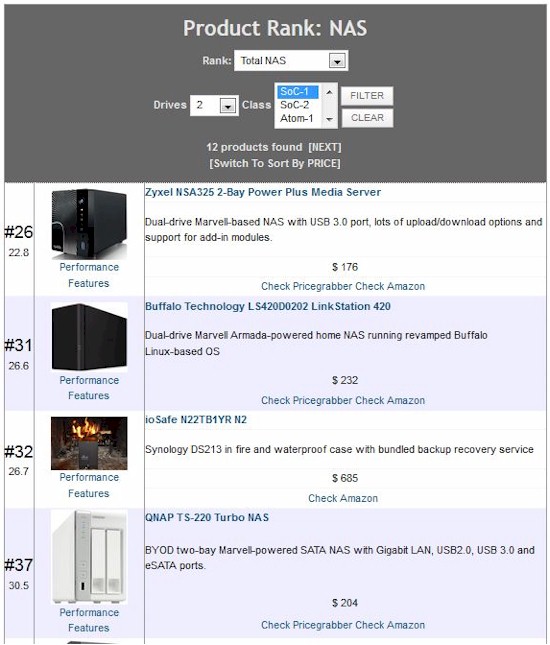The image displays a graphical user interface, specifically a search and filter window for network-attached storage (NAS) products. The top section of the window has a gray header titled "Product Rank NAS". Below this title, there are various interactive input fields and dropdowns. 

- The first input box is labeled "Rank" and displays "Total NAS."
- The next section, titled "Drives," shows the number 2.
- Below that, a "Class" dropdown menu contains options: SOC 1, SOC 2, and Atom 1, with SOC 1 currently highlighted.
- Further down, there are two buttons labeled "Filter" and "Clear."

Below these controls, the interface indicates "12 products found" with a "Next" button adjacent to it, suggesting pagination for additional results. Below this, there is an option to "Switch to sort by price."

The product list starts with a detailed item entry:
- The top-ranked item, numbered 26, is the "ZYXEL NSA325 2-Bay Power Plus Media Server." It features dual drives, a marvel-based NAS, a USB 3.0 port, numerous upload/download options, and support for add-in modules, priced at $176.

Following entries include:
- "Buffalo Technology LinkStation 420" priced at $232.
- "IO Safe," priced at $685.
- "QNAP TS-22 Turbo NAS," priced at $204.

The displayed rankings for these NAS products are 26th, 31st, 32nd, and 37th, respectively. Each product entry includes performance features and additional specifications where relevant.